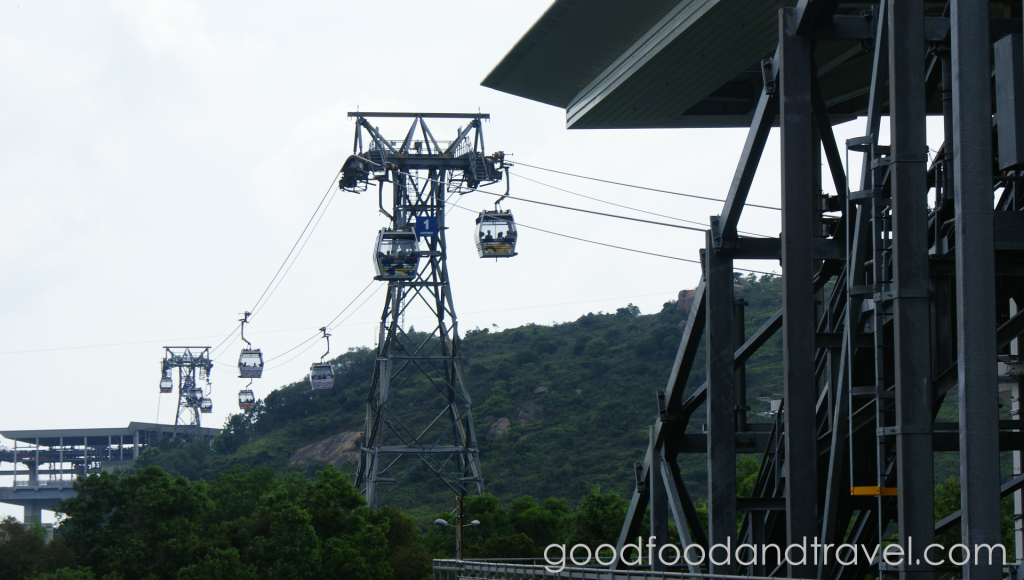The image depicts a cable car ride resembling a ski lift, potentially similar to those found at Disney World. Taken from the perspective of a station, the scene shows a total of eight cable cars suspended on cables, traveling between two towers. There are two platforms visible—one in the foreground and another in the background. The landscape features lush greenery with an abundance of trees and a cloudy, grey sky. Superimposed text on the image reads, "protect more of your memories for less," and at the bottom right corner, there's the website "goodfoodandtravel.com." Additionally, a barely visible Photobucket watermark, consisting of a series of concentric circles, is present in the center.